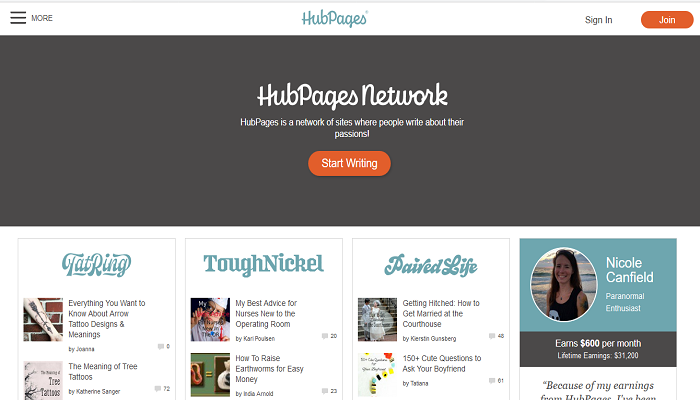The image displays a web page with a clean, white background. At the center, "HubPages" appears prominently in blue text. Across the top of the page, there are various navigation options, including a "Sign In" link and an orange "Join" button. To the left, there is a menu indicator marked by the word "More" accompanied by three horizontal lines. A gray banner runs across the page, featuring white text that reads "HubPages Network." This section describes HubPages as a network of sites where individuals can write about their passions. Below the banner, there's another orange button labeled "Start Writing."

Towards the bottom of the page, several sections of content are displayed, each varying in font style and size. "TatRing" is presented in a decorative font, offering information about arrow tattoo designs and their meanings, as well as the significance of tree tattoos. In the center, the name "ToughNickel" is written in a notable blue font, accompanied by article titles such as "My Best Advice for Nurses New to the Operating Room" and "How to Raise Earthworms for Easy Money."

Adjacent to these entries, "PairedLife: Getting Hitched" features articles like "How to Get Married at the Courthouse" and "150+ Cute Questions to Ask Your Boyfriend." Additionally, there is a small photo of Nicole Canfield, who is identified as a paranormal enthusiast. The entire layout is designed to be user-friendly, guiding visitors towards content that matches their interests and encouraging them to contribute their own writings.